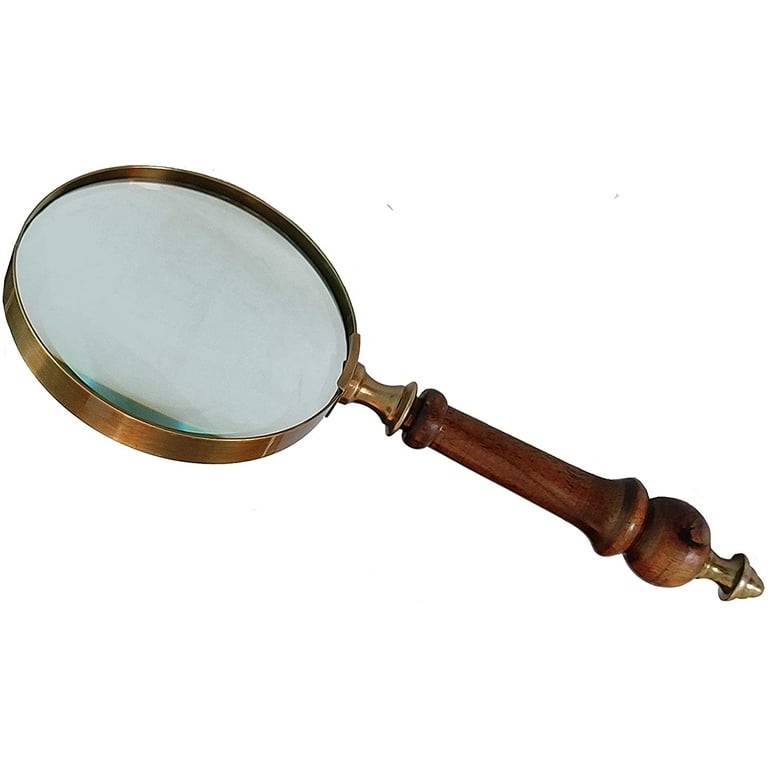This photograph captures an exquisitely detailed, antique magnifying glass that evokes a sense of Victorian elegance, reminiscent of a Sherlock Holmes novel or classic detective films. The magnifying glass is quite large, yet comfortably holdable with one hand. Its handle is made of dark brown, polished wood, oiled and lacquered to a glossy shine, and features a brass knob at the bottom, adding a touch of decorative sophistication. The circular lens is encased in a brass frame with a slightly golden hue, giving it a rich antique character. The glass itself, though clear, exhibits a subtle bluish tint and appears aged, possibly dust-covered, hinting at years of use or idle display. This beautifully crafted piece is set against a stark white background, ensuring its every detail stands out, highlighting its dual nature as both a functional tool and an artful decorative object.